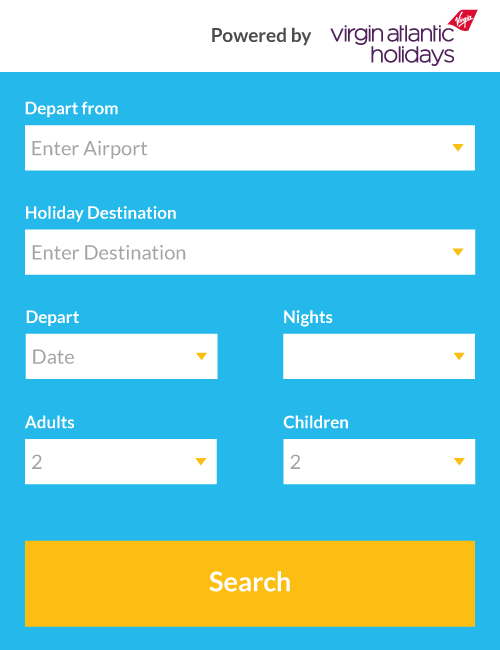The image showcases a search screen designed for travel planning. At the top, a prominent white banner displays text in black reading "Powered by," followed by a slightly larger font stating "Virgin Atlantic Holidays" along with the recognizable red Virgin logo positioned at the top right corner. The screen features a blue background that contains a series of white fields intended for conducting a detailed search.

The first field is labeled "Depart From," allowing users to select their departure airport via a dropdown menu. Directly below it is the second field labeled "Holiday Destination," where users can choose their desired destination, also through a dropdown menu. Positioned to the left beneath these two fields, users will find options to specify the "Departure Date" and the duration of their stay denoted as "Nights," both with dropdown menus for easy selection. 

Further down, the form lets users customize their travel party by adjusting the number of "Adults," which has a default value of two, and the number of "Children," also set to a default of two; both of these values can be changed using the provided dropdown options.

At the bottom of the search fields, a large, eye-catching yellow button with bold white text reads "Search," prominently indicating the action users should take after entering their travel criteria. Once all necessary information is filled out, clicking this button will initiate the search process based on the specified parameters.